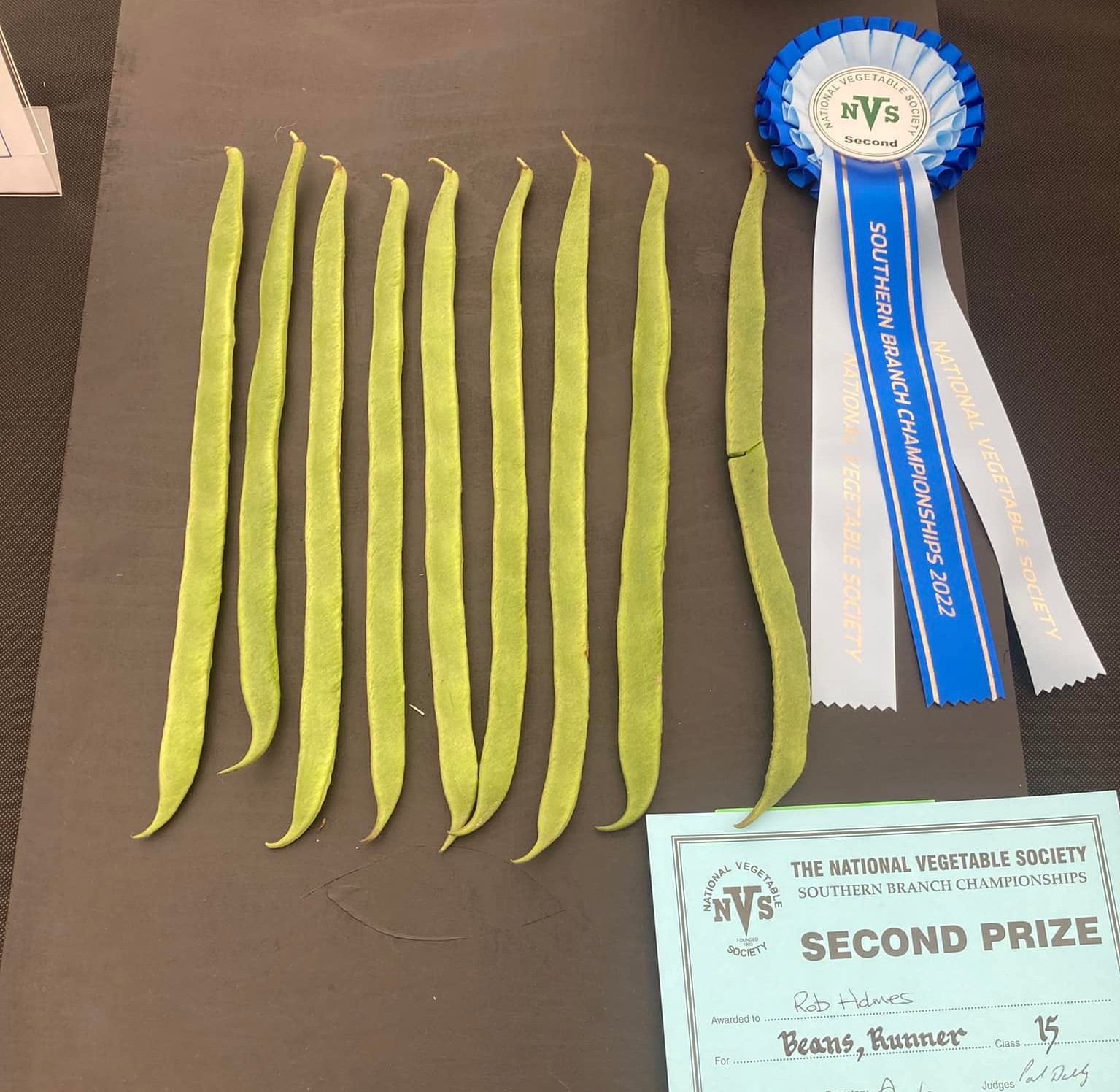The photograph captures an award-winning display of nine long, healthy runner beans laid out on a dark brown or black surface. To the right, a blue ribbon prominently showcases the text "NVS" (National Vegetable Society) and "Southern Branch Championships 2022." Beneath the ribbon, there is an engraved certificate, proclaiming it the second prize winner at the National Vegetable Society Southern Branch Championships. The certificate further details that the award was given in the category of beans, specifically runner beans, class 15, and was presented to Rob H. D. M. E. S. A small green sheet of paper with signatures is partially visible beneath the certificate. The collection of pristine and vibrant beans, with one slightly imperfect specimen, underscores the accomplishment celebrated by this award.